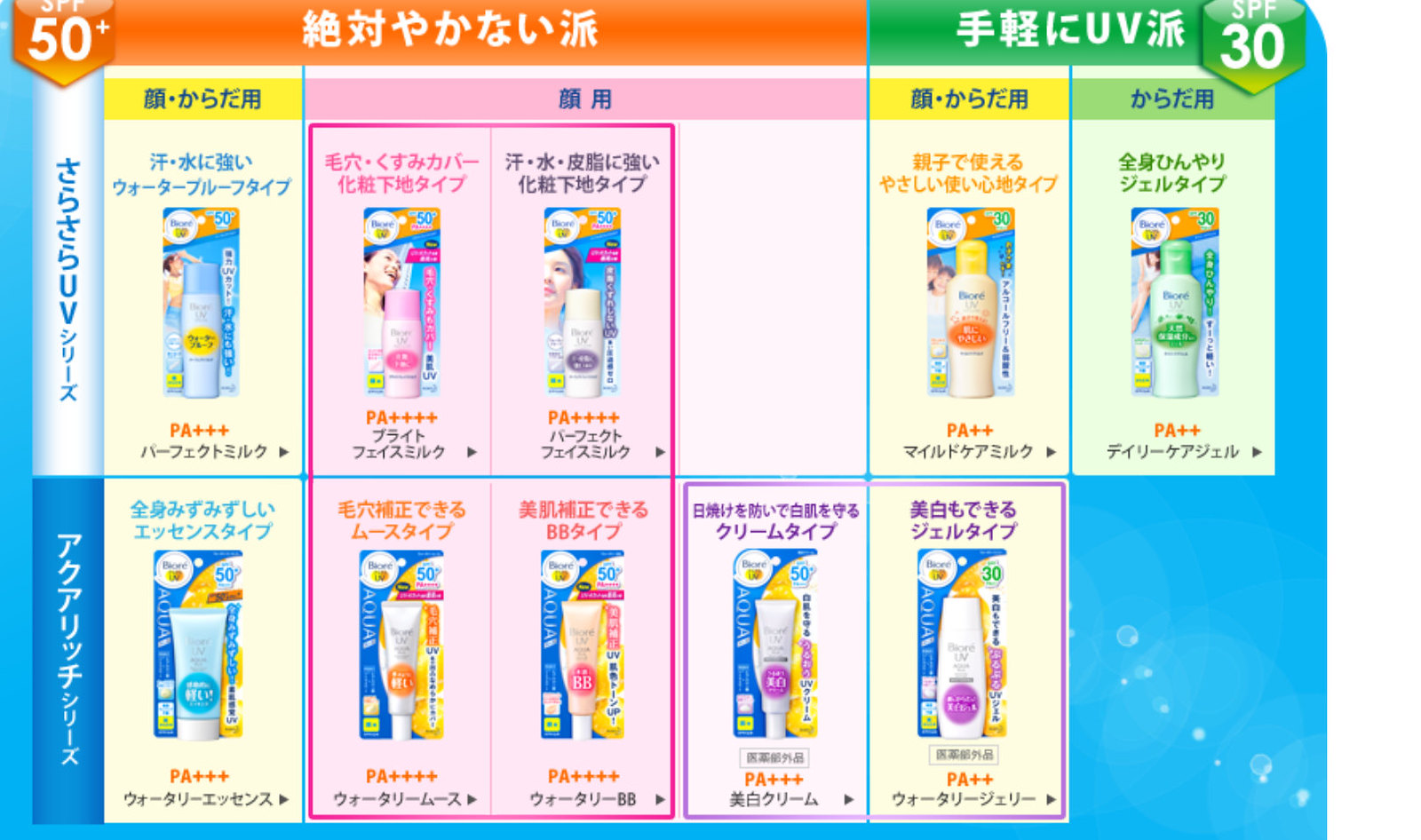The image is an advertisement in Japanese, showcasing a variety of sunscreen products. The entire background is light blue, with a decorative element of bubbles in the bottom right corner. The layout consists of a grid featuring two main rows of sunscreen bottles. Each column in this grid is color-coded: yellow, pink, green, and blue, with a mix of different sunscreen bottles in each.

At the top left corner, it indicates SPF 50+ with an orange border, and at the top right corner, it indicates SPF 30 with a green border. The bottles vary in size and shape, resembling miniature shampoo bottles or travel-size packages. 

In the first column, both the top and bottom bottles are yellow. The next three columns are primarily pink, but the arrangement leaves one spot blank in the top row. The fifth column is green, containing a bottle on the top row, while the rest below it is blue. Notably, the bottles are numbered, predominantly showing "50," which hints at their SPF rating.

The bottles depict various scenarios: one features an Asian woman smiling and looking upwards, another shows only half her face looking left, yet another features a mother and daughter touching faces and smiling, and one has a woman touching her legs. Smaller tube-like bottles with caps, bearing the letters "BB," are also visible in the bottom row, likely indicating beauty-related products.